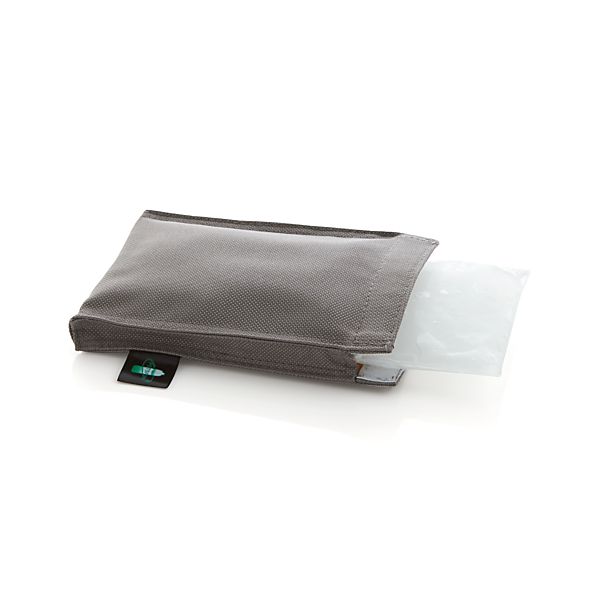This image features a small, gray, stitched fabric pouch with a high-quality appearance and an open end. A clear plastic packet, resembling a bag of ice or a placeholder to maintain the pouch's shape during shipping, protrudes from the right side. The pouch seems to have a magnetic closure, indicated by a silver segment at the bottom right. A black tag with an image resembling a green and white bullet is attached to the lower left corner. The entire scene is set against a plain white background.